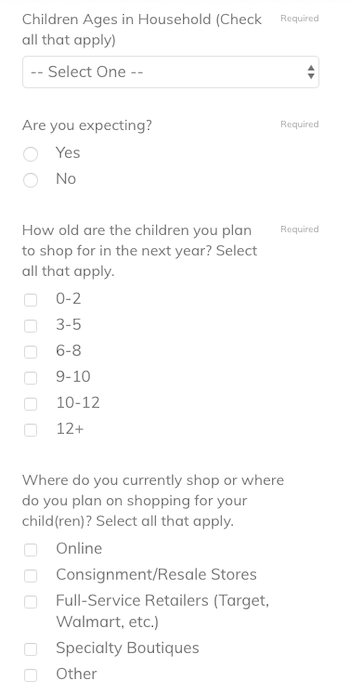Upon close examination, the image appears to be a screenshot from a mobile device displaying a survey with demographic questions. The text is set in black on a white background. Here's a detailed breakdown:

- The first question asks: "Children ages in household (check all that apply)." There is a drop-down menu labeled "Select one," which likely contains a list of age ranges. This field is marked as "required" in gray text.
- The next question is: "Are you expecting?" There are two checkboxes provided for "Yes" or "No," and this question is also indicated as "required."
- Following that, another question reads: "How old are the children you plan to shop for in the next year? (Select all that apply)." The available checkboxes are for the age ranges: 0-2, 3-5, 6-8, 9-10, 10-12, and 12+. This question is also marked as "required."
- The final question asks: "Where do you currently shop or where do you plan on shopping for your child(ren)? (Select all that apply)." The provided options with checkboxes include: Online, Consignment/Resale Stores, Full-Service Retailers (e.g., Target, Walmart), Specialty Boutiques, and Other. No checkboxes are checked for this question.

This detailed description encapsulates all visible elements of the survey, ensuring clarity and completeness.